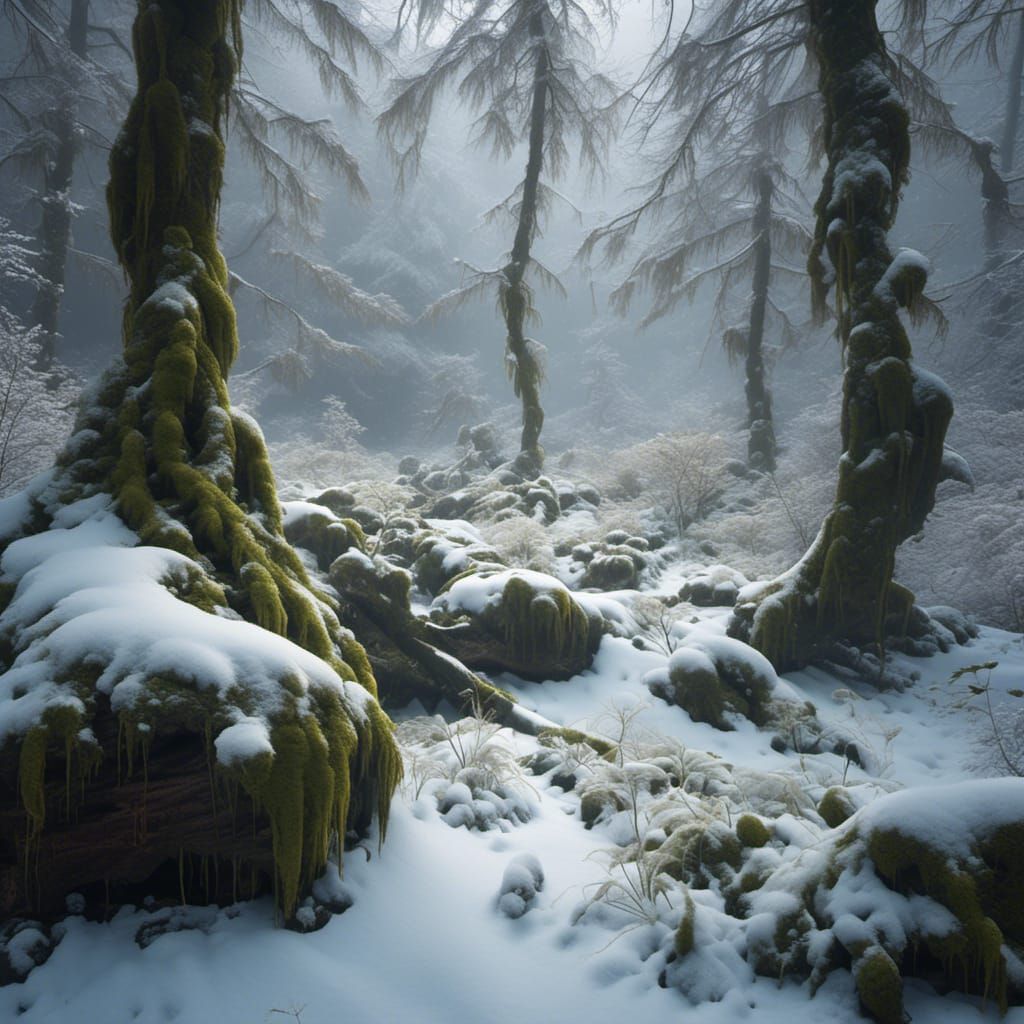In this detailed, fantasy-like winter scene, the photo captures a snow-covered forest featuring gnarly, spindly trees with needle-like leaves rather than typical foliage. These trees appear almost mystical, as their bark and long, twisted roots are cloaked in a draping green moss that seems to hang like liquid strands, adding to their fantastical appearance. The snowy ground is rough and uneven, with bulbous shapes and protruding roots suggesting hidden rocks beneath the surface. 

A large rock formation, heavily blanketed in both moss and snow, stands prominently on the left side of the image, with a tree rising from behind it, also adorned in moss. The entire forest floor is thickly layered in white snow, integrating rocks and any underlying greenery into the wintry tableau. In the distance, other trees, resembling tall pines, extend endlessly, their forms shrouded in muted grays, browns, and greens with only a hint of light peeking through the dense foliage. This muted color palette, combined with the textural interplay of moss and snow, creates an enchanting, otherworldly atmosphere.